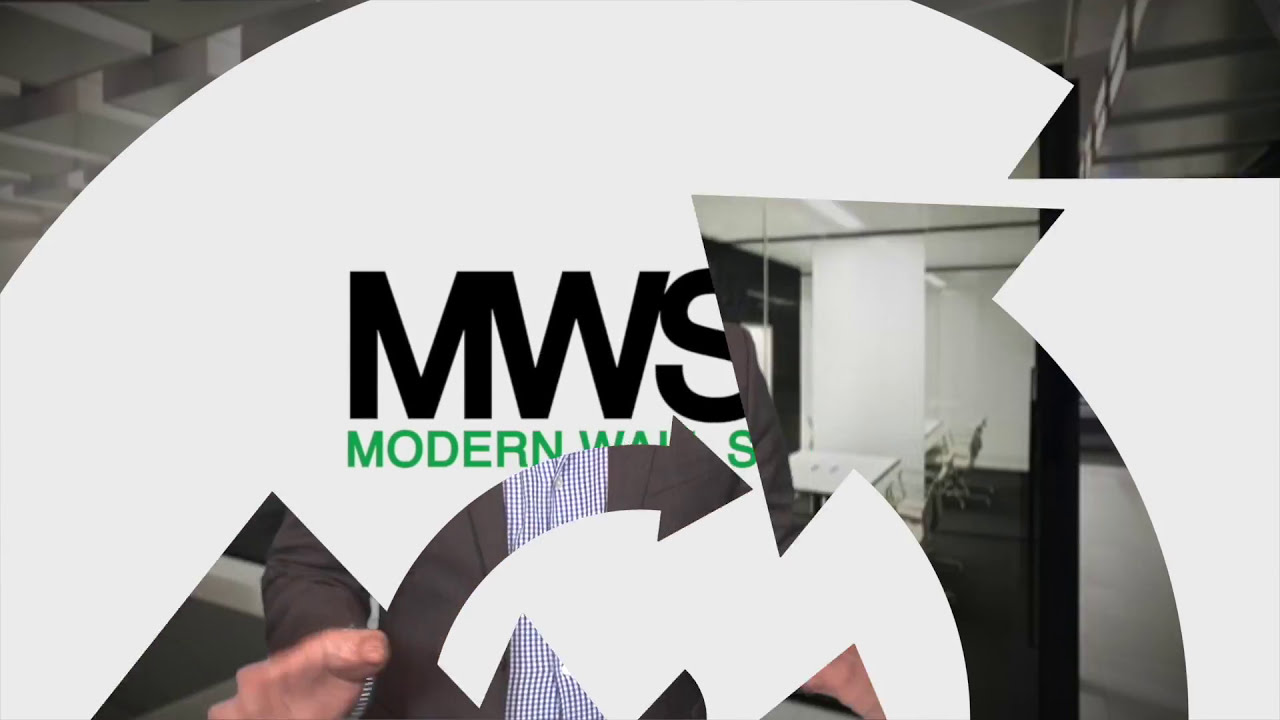The horizontal rectangular image appears to be an advertisement for a company, featuring a sophisticated design. Abstract white arrows and arcs, some solid and some cutouts, overlay a blurred background showing parts of a room with white walls and black cabinets, possibly an office environment with a flight of stairs. In the center, bold black letters spell out "MWS," likely in a Helvetica-type font. Beneath "MWS," green text partially reads "modern," though the full phrase is obscured, suggesting movement or an animation effect. On the bottom left, a man's hand, possibly belonging to someone in business casual attire, holds a tool, adding a dynamic element to the scene. The intricate white designs and partially visible background create a sense of motion and depth, aligning with the ad's modern, professional theme.